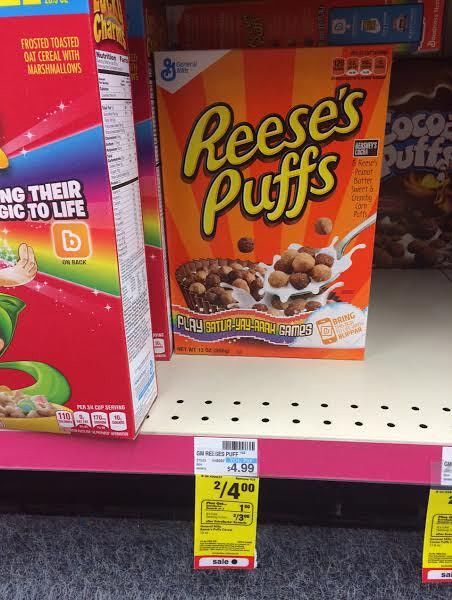This photograph captures a well-stocked grocery store shelf prominently featuring a variety of cereals. The main focal point of the image is a box of Reese's Puffs cereal, which stands out with its distinct branding reminiscent of a Reese's Peanut Butter Cup. The Reese's Puffs logo is displayed in bright yellow letters, set against a vibrant orange background. Below the logo, an image depicts the cereal, designed to appear as though it is inside a Reese's cup, acting as a bowl. The visual includes a spoon emerging from the right side, dipping into the milk-filled cereal, suggesting someone is about to enjoy a delicious breakfast.

Adjacent to the Reese's Puffs, on the left side, a partial view of a Lucky Charms cereal box is visible. Distinctive elements such as the colorful rainbow arch and the iconic red background of the Lucky Charms box can be seen, adding to the vibrant display. A bright yellow sale tag catches the eye, announcing a promotional offer: "Two for Four Dollars," marked down from the regular price of $4.99. The sale tag features contrasting colors of yellow, red, and white, making it easily noticeable against the white price tag background.

Overall, this detailed snapshot highlights the enticing cereal options available on the grocery store shelf, with a special emphasis on the visually appealing Reese's Puffs cereal box and the attractive sale offer.